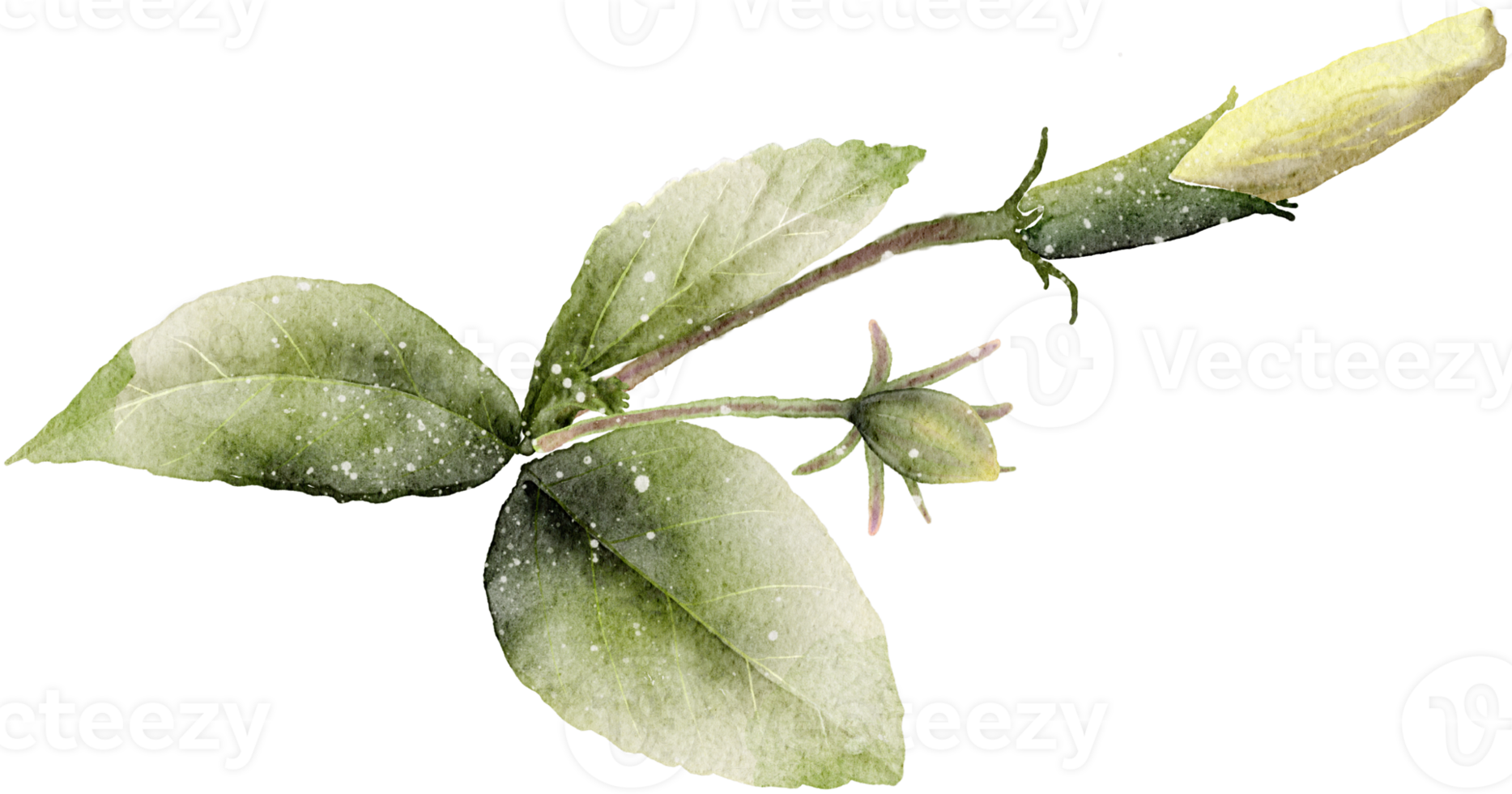This image features a lush close-up of a plant, depicted in a watercolor style against a completely white background. Dominating the foreground are three pointed green leaves, each showcasing varying shades of medium to light green with delicate white splotches that add texture and detail. Two brownish stems extend from the plant, one bearing an unopened whitish-yellow flower bud and the other supporting a less mature, oval-shaped pod surrounded by spiky protrusions. Both buds are oriented toward the right side of the image. The composition is heavily processed, resulting in a stylized, almost painting-like appearance, overlaid with the watermark “Vecteezy” and an ornate “V” icon, scattered throughout the entire image.